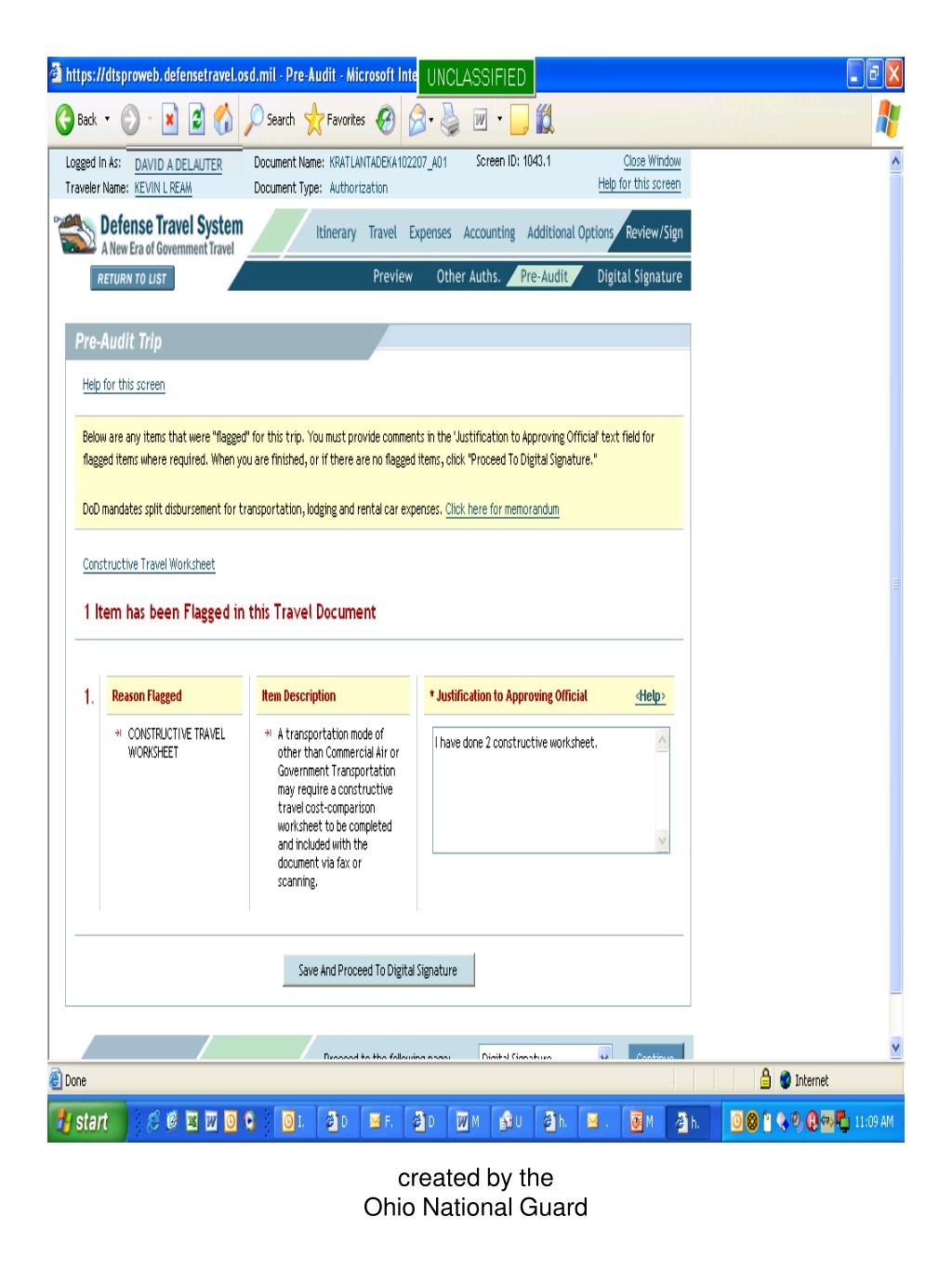**Caption: Screenshot of an Old Microsoft Defense Travel System Interface**

This screenshot captures the interface of an old Microsoft application, specifically the Defense Travel System (DTS). The layout includes multiple segments that detail various features and processes within the system. The main focus is on a pre-audit trip help screen. 

In the central panel, there is a notification describing the need for comments in the "justification to proving official" text field for any flagged items. Users are required to address these flagged items before proceeding. The document mandates specific discernment for transportation, lodging, and rental car expenses by the Department of Defense (DoD).

One item, related to a "constructive travel worksheet," has been flagged. The text indicates that in certain cases, a cost comparison worksheet for transportation must be completed and included via fax or scanning. Additionally, user comments indicate the completion of two constructive worksheets, although it remains unclear why the item was flagged.

The interface layout includes buttons for navigation such as 'Back,' 'Delete,' 'Return,' 'Home,' 'Search,' and 'Favorites.' An 'Email' option is also visible, hinting at integration with a Microsoft email inbox.

Overall, this screenshot provides a glimpse into the operational details and user interface of the historical Defense Travel System used for managing and approving travel-related expenses for DoD personnel.